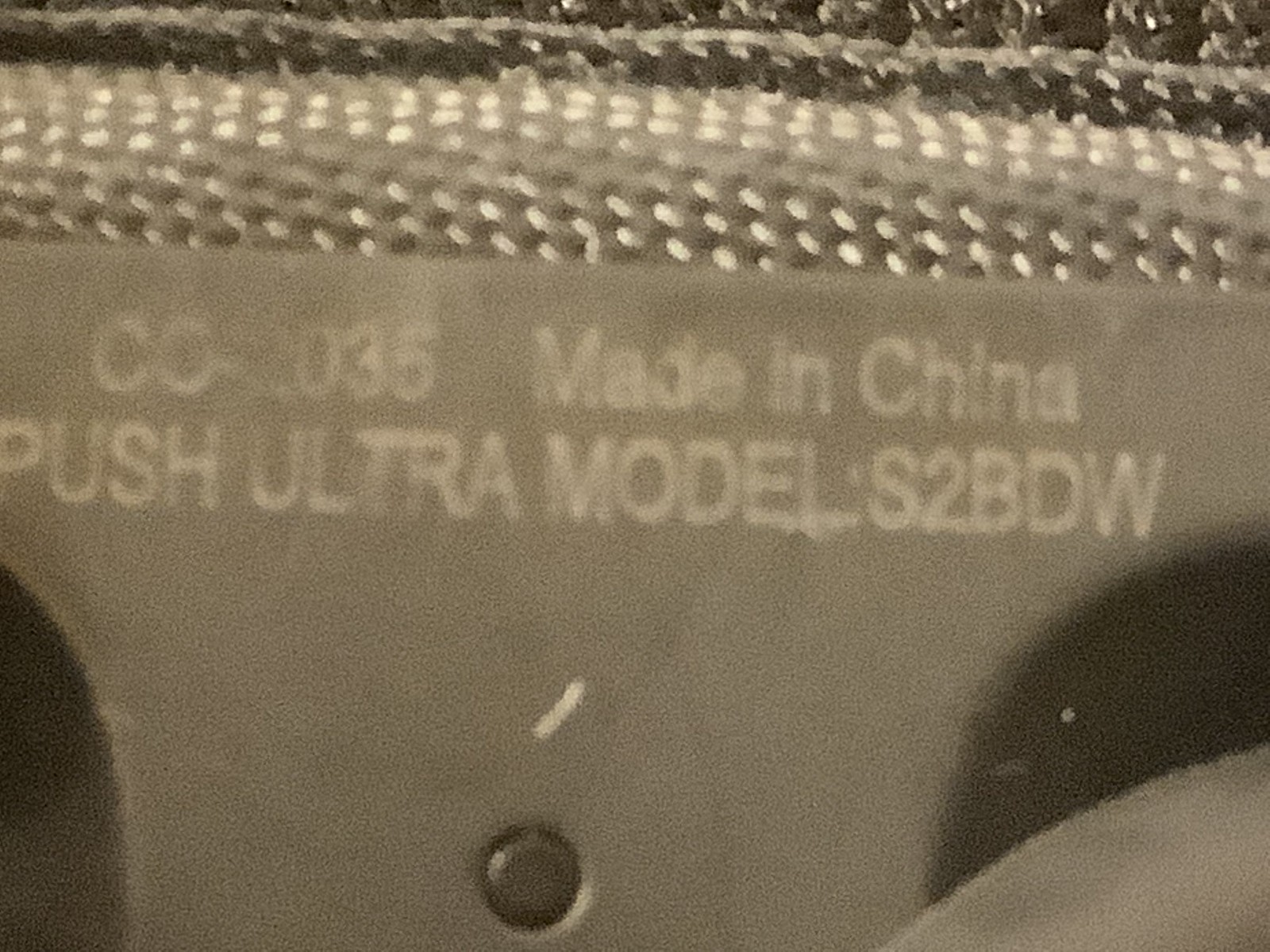The image features a close-up of what appears to be an early piece of technology, potentially the back of a cassette tape or a woven fabric item like a purse or shoe. The central upper part of the image showcases a horizontal strip of silver mesh material spanning from the left to the right edge. Below this strip, the background is a tannish gray color with distinctive white text that reads "CO2035 made in China Push Ultra Model S2BDW." Centered in the middle area, there is a dark gray button, flanked by two large black circles suggestive of the reels of a cassette tape. Additionally, there is a small white mark beneath the text and a round plastic circle is noticeable in the lower section of the image. The entire composition sits against a completely gray backdrop.